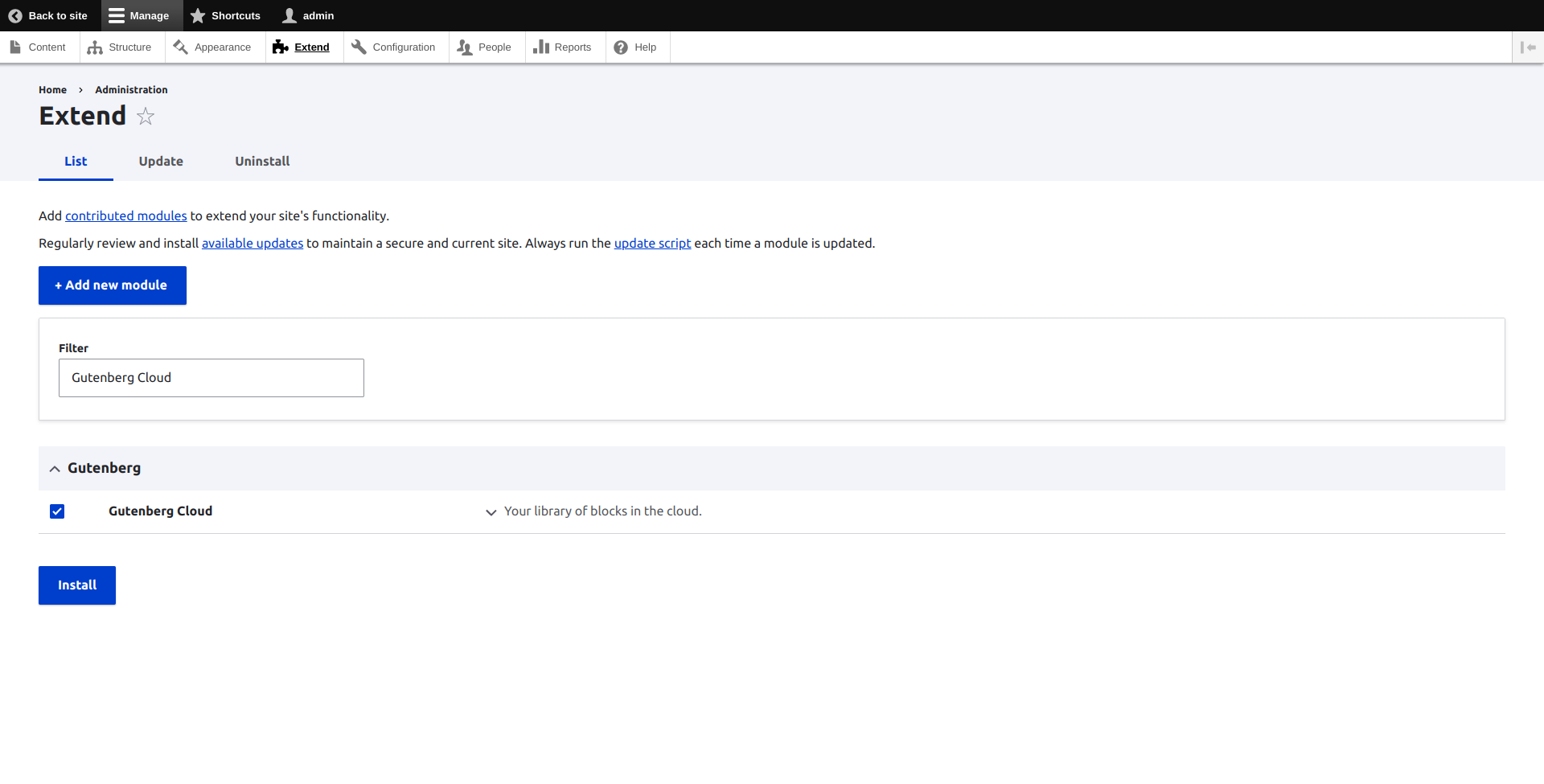The image displays a webpage interface with a black header at the top, followed by a white header underneath. Below the headers, there are several menu options listed in a structured layout:

1. **Black Header**
   - Not specified

2. **White Header**
   - Contains multiple sections including:
     - **Content**
     - **Structure**
     - **Appearance**
     - **Extend (Configuration)**
     - **People**
     - **Reports**
     - **Help**

3. **Main Menu Options (Below Headers)**
   - The "Extend" option is highlighted in a darker shade to indicate it is currently selected.

4. **Sub-menu Under "Extend"**
   - Home
   - Administrative
   - List (Highlighted in blue)
   - Update
   - Uninstall

5. **Descriptive Text**
   - The screen provides instructions and additional information relevant to the "Extend" section:
     - "Add contributed modules to extend your site's functionality." The phrase "contributed modules" is highlighted in blue, indicating it's likely a hyperlink.
     - "Regularly review and install available updates to maintain a secure and current site. Always run the update script each time a module is updated." Both "update script" and "available updates" are in blue, suggesting they are also hyperlinks.

Overall, the image portrays a detailed and interactive webpage focused on managing and extending a website's functionality through modules, updates, and configurations.